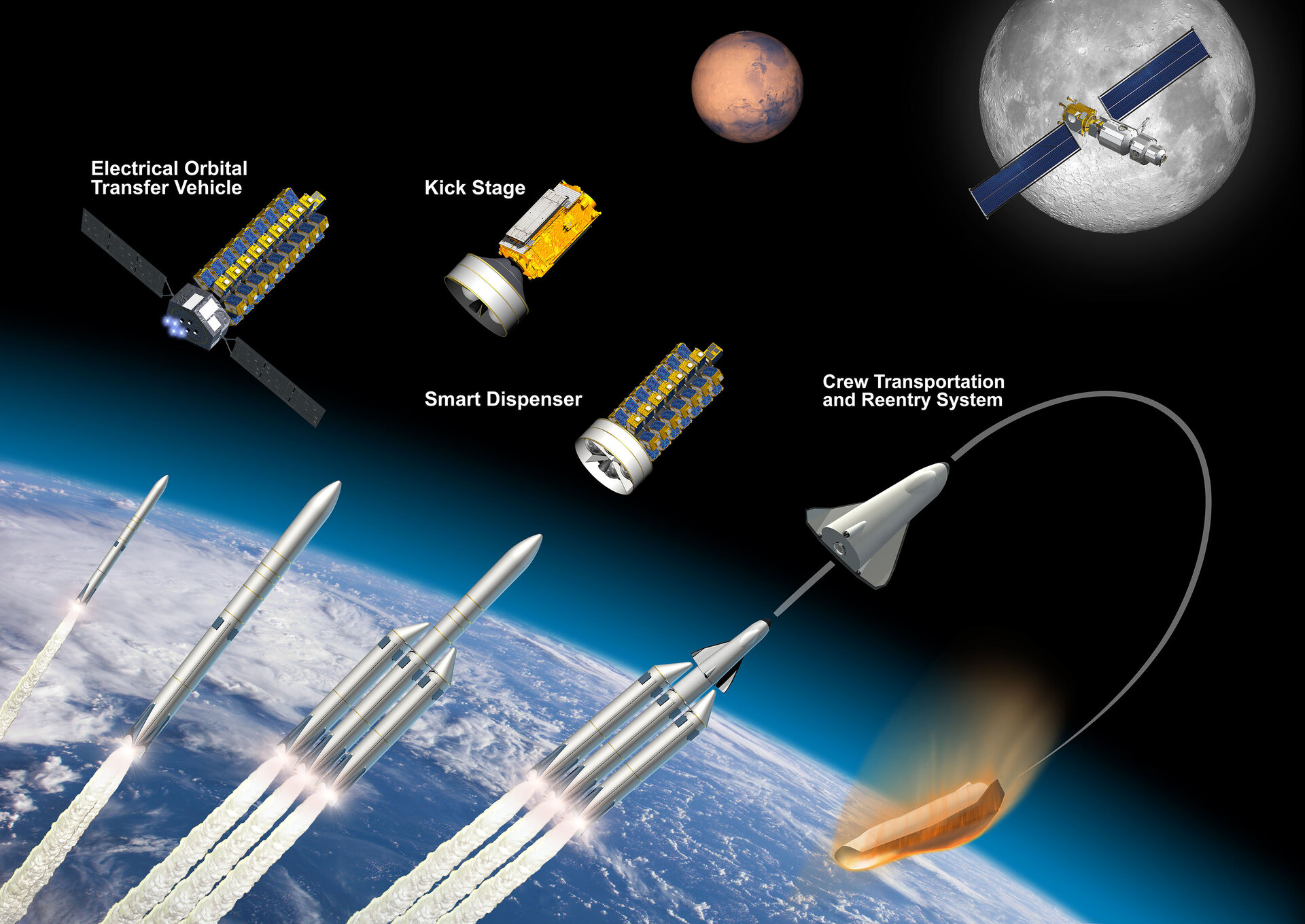The image is a detailed diagram of space shuttle systems and their associated components, set against the backdrop of outer space just outside Earth. The Earth is prominently visible, showing its blue oceans and white atmospheric layers, transitioning into the blackness of space. The moon can be seen in the top right, Mars in the top middle, and several satellites are scattered around the scene. Key elements in the diagram include the Electrical Orbital Transfer Vehicle, Kickstage, Smart Dispenser, and Crew Transportation and Reentry System, each accompanied by corresponding illustrations. The various colors used—blue, white, orange, red, black, yellow, and hints of green and brown from Earth—suggest a professional, educational illustration aimed potentially at school children or for general educational purposes. This chart effectively explains different stages of a rocket's journey and its components, with detailed textual labels in white providing further explanations. A large telescope-like satellite is foregrounded against the moon, illustrating the educational intent of the image.